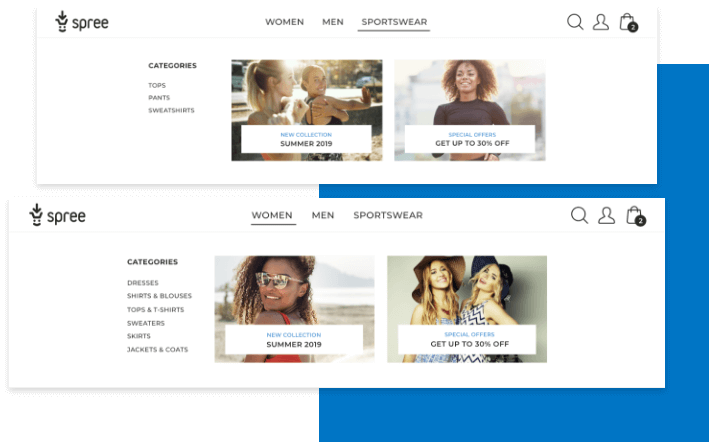A detailed screenshot of a website named "Spree" displays its Clothing for Sale utility interface, featuring two similar but distinct sections. Both sections are horizontally elongated white rectangles, each containing navigation elements and promotional images.

At the top section, the highlighted "Sportswear" tab is underlined, indicating the current category selection. The navigation bar, consistent across both sections, displays "Spree" on the left, with links to "Women's," "Men's," and "Sportswear" categories in the middle. To the right of the navigation bar are icons for search, user account, and a shopping bag with a notification of two items.

The Sportswear section lists categories on the left, including "Categories," "Tops," "Pants," and "Sweatshirts." Two promotional images are presented: one marked "New Collection, Summer 2019," and another stating "Special Offers get up to 30% off."

The lower section shows the "Women's" category tab as the currently selected option. On the left, categories listed include "Categories," "Dresses," "Shirts and Blouses," "Tops and Shirts," "Sweaters," "Skirts," and "Jackets and Coats." Similar to the Sportswear section, this area features the same promotional images with identical captions: "New Collection, Summer 2019," and "Special Offers get up to 30% off."

Both sections are outlined against a larger blue square background on the right, with only the right portion of the white rectangles overlaying it, creating a visually distinct composition. The overall color palette predominantly includes white, blue, black, and gray.